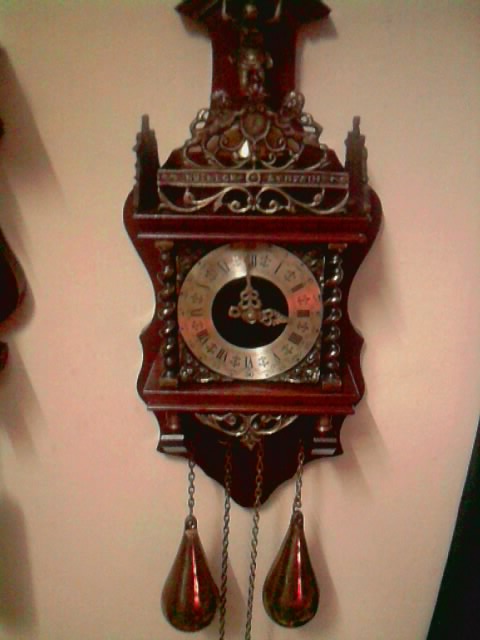This photograph showcases a beautifully ornate, wall-mounted grandfather clock set against an off-white backdrop. The clock’s body is crafted from rich mahogany wood, giving it a striking reddish-brown hue. The design of the clock resembles an upside-down acoustic guitar, with an hourglass-like curved silhouette. The top section features elaborate metalwork that resembles a crown flanked by wooden pillars, adding to its regal appearance.

The clock’s face is silver, adorned with Roman numerals, and is encircled by intricate black detailing. The elegantly carved hour and minute hands point to 2:59. Below the clock face, there are two teardrop-shaped counterweights suspended from chains, alongside additional chains extending below the frame, hinting at its wind-up mechanism.

Adding to its complexity are detailed engravings, including what appears to be a humanoid figure accompanied by two big cats on their hind legs, contributing to the clock’s ancient and sophisticated design. Overall, this clock is a stunning blend of detailed craftsmanship and timeless elegance.